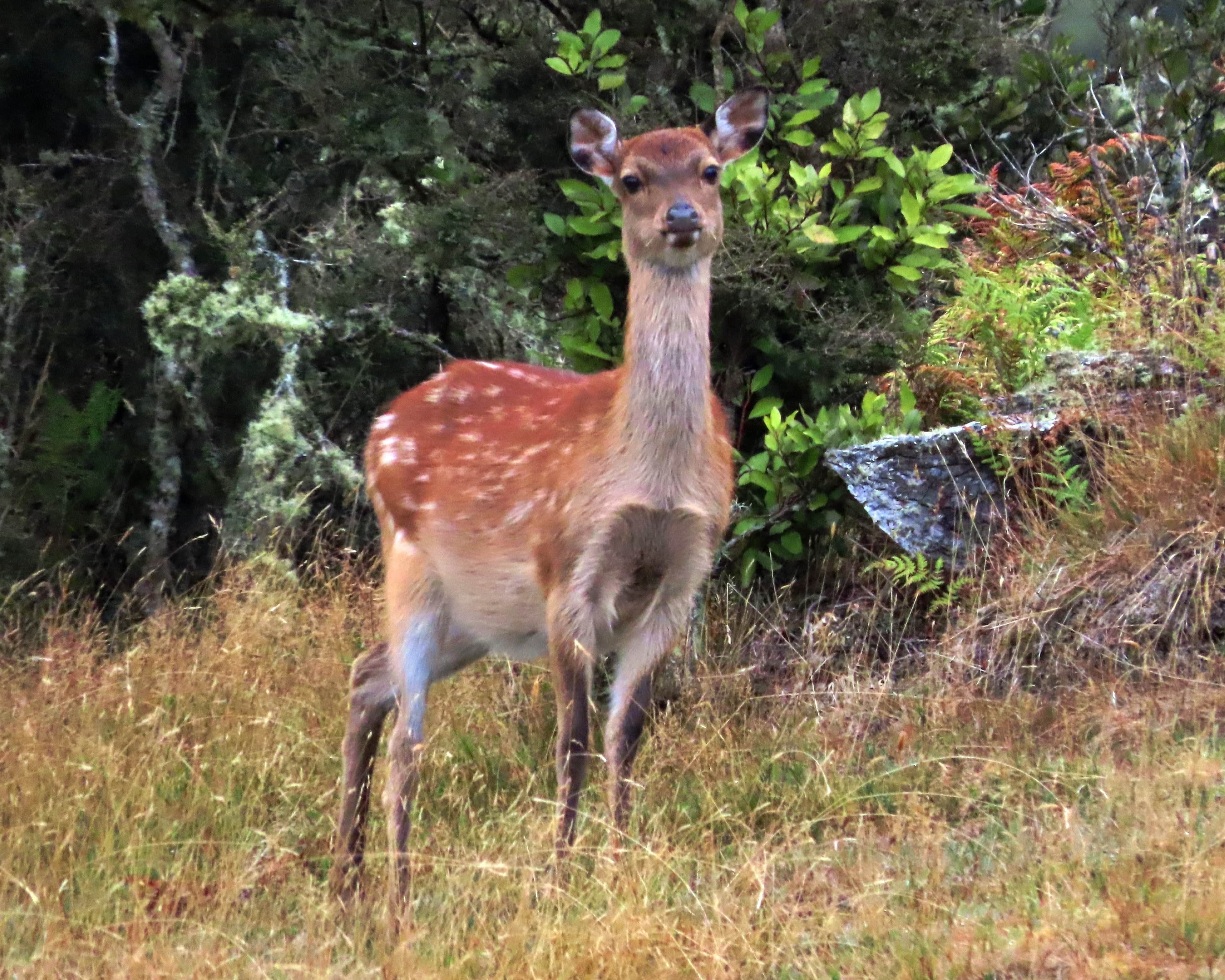This is an image of a young deer standing alert in a grassy field, surrounded by various shades of green and brown vegetation. Its slender legs support its graceful body, covered in brown fur with distinctive white speckled markings. The deer's ears are perked up, suggesting it is listening intently, and it gazes directly at the camera with its black eyes and black nose. In the background, the setting transitions into a dark, dense forest, creating a striking contrast to the brighter green plants and rocks scattered around the deer's immediate vicinity. The tall grass it stands in is a mixture of green, brown, and a hint of yellow, while a large rock and additional shrubbery add to the natural scenery. Despite the photographic quality, there is a subtle artistic, almost painted, feel to the image, enhancing the deer's serene presence in its lush, detailed environment.